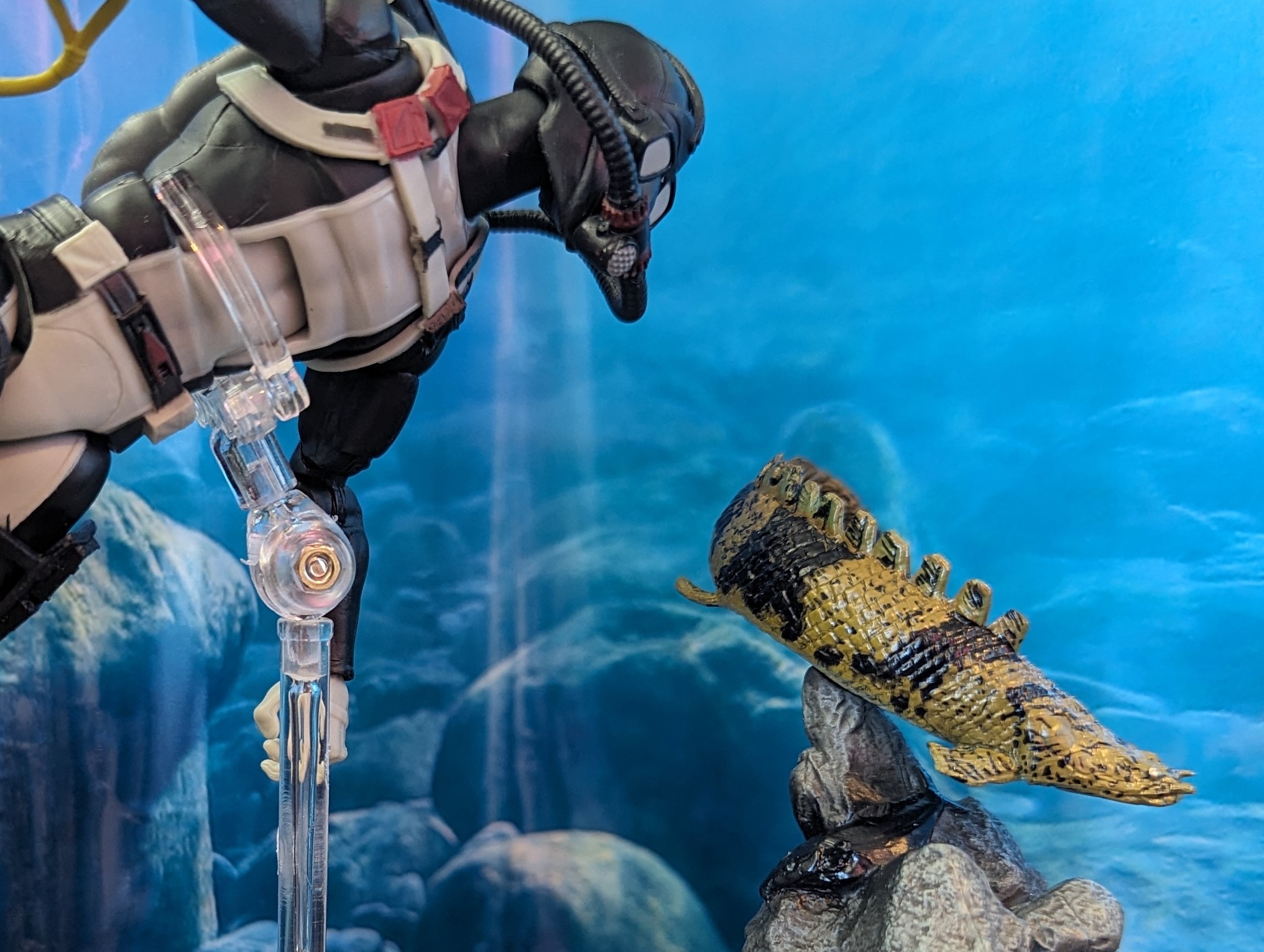In this underwater scene, a scuba diver, donned in a black wetsuit with a gray front and a white overlay, navigates the deep blue sea. The diver, who wears a black helmet and black goggles, holds a clear tubular apparatus pointed downward with his right hand while his other hand is outstretched behind him. Strapped to his back is a tank, and a clear device wraps around his waist, possibly indicative of a specialized tool or component. The seabed, covered with large rocks, forms the backdrop amidst the vibrant cobalt water. On the right side, the diver's attention is captured by a peculiar, golden fish adorned with dark stripes and a series of pointed fins along its body, giving it a somewhat snake-like, eel-shaped appearance with bumpy scales. The fish, appearing almost fantastical, suggests a mixture of browns, tans, and reds, contributing to a scene rich in color and mystique. The realistic elements combined with the unusual features of the fish give the image an almost surreal, possibly AI-created quality.